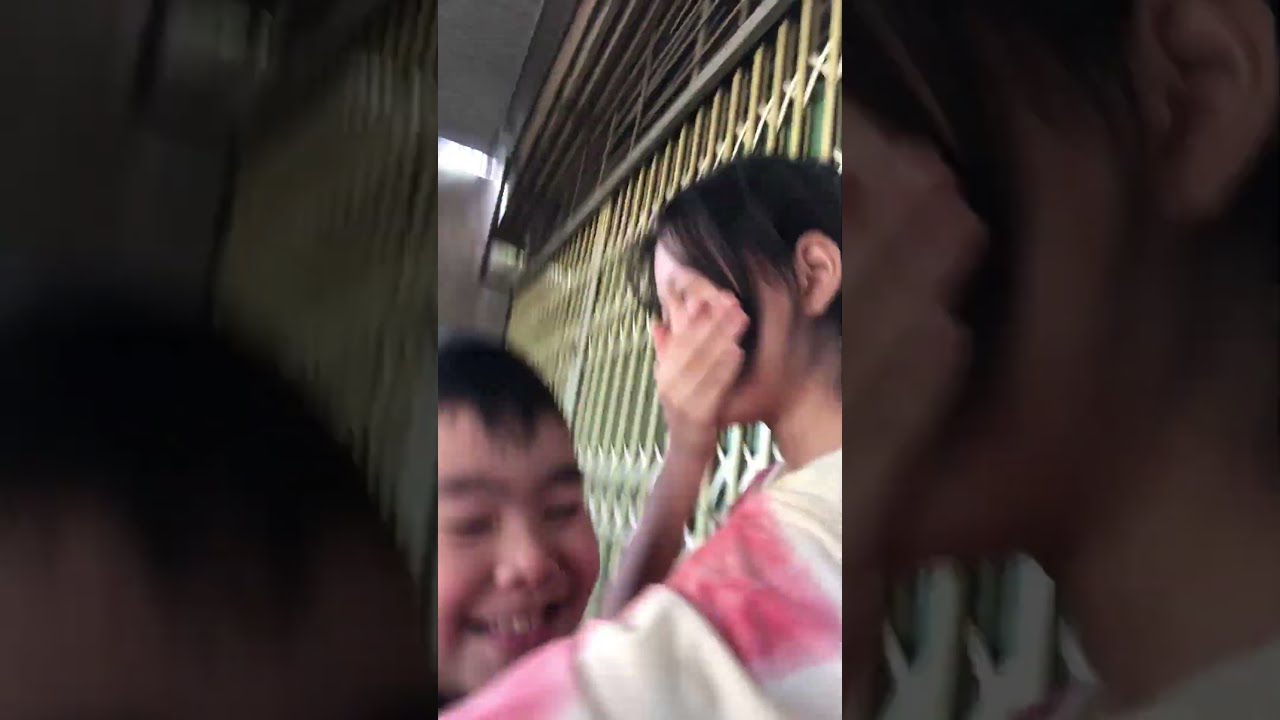The photograph captures a candid moment between two people, slightly blurry and taken from a camera phone. Dominating the center, a young man with short black hair and thick eyebrows, possibly of Asian descent, is smiling with his eyes closed. He appears to be genuinely happy, likely laughing. To his right, a young woman, slightly taller, also with black hair swept up with bangs framing her face, is laughing as well. She is covering her mouth with one hand, suggesting she's trying to hold in a joke. The woman's attire consists of a white shirt with pink accents. They both stand in front of what seems to be a metal gate, possibly an elevator gate or a gate like those found at store entrances in malls. The image background gives a sense of depth with slightly blown-up and shadowed borders.